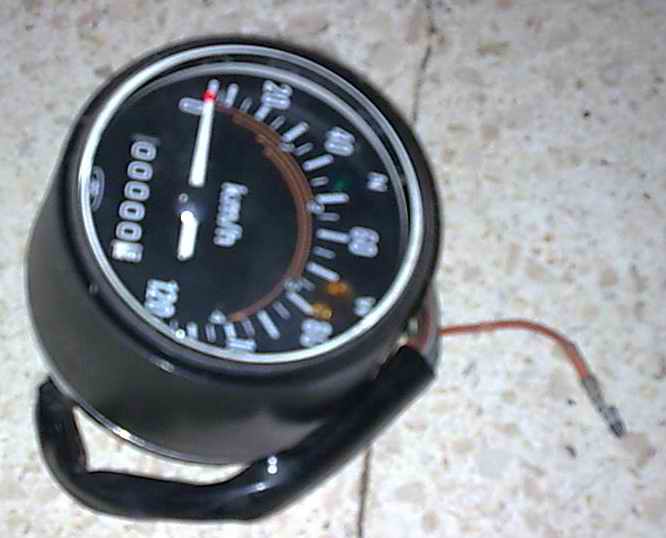On a polished marble surface lies a speedometer, positioned sideways with its bottom oriented to the left. The speedometer measures speeds from 0 to 120 kilometers per hour. Its face is black, contrasting sharply with the white numbering and pointers. The needle, featuring a red dot at its tip, points towards the scale. Below the dial, the odometer section displays a series of zeros (000000), indicating that no mileage has been accumulated. The blurred image highlights several wires protruding from the back of the speedometer, designed to connect to a vehicle, likely a scooter or motorcycle based on the speed range. Among the tangle of wires, one stands out distinctly in red.